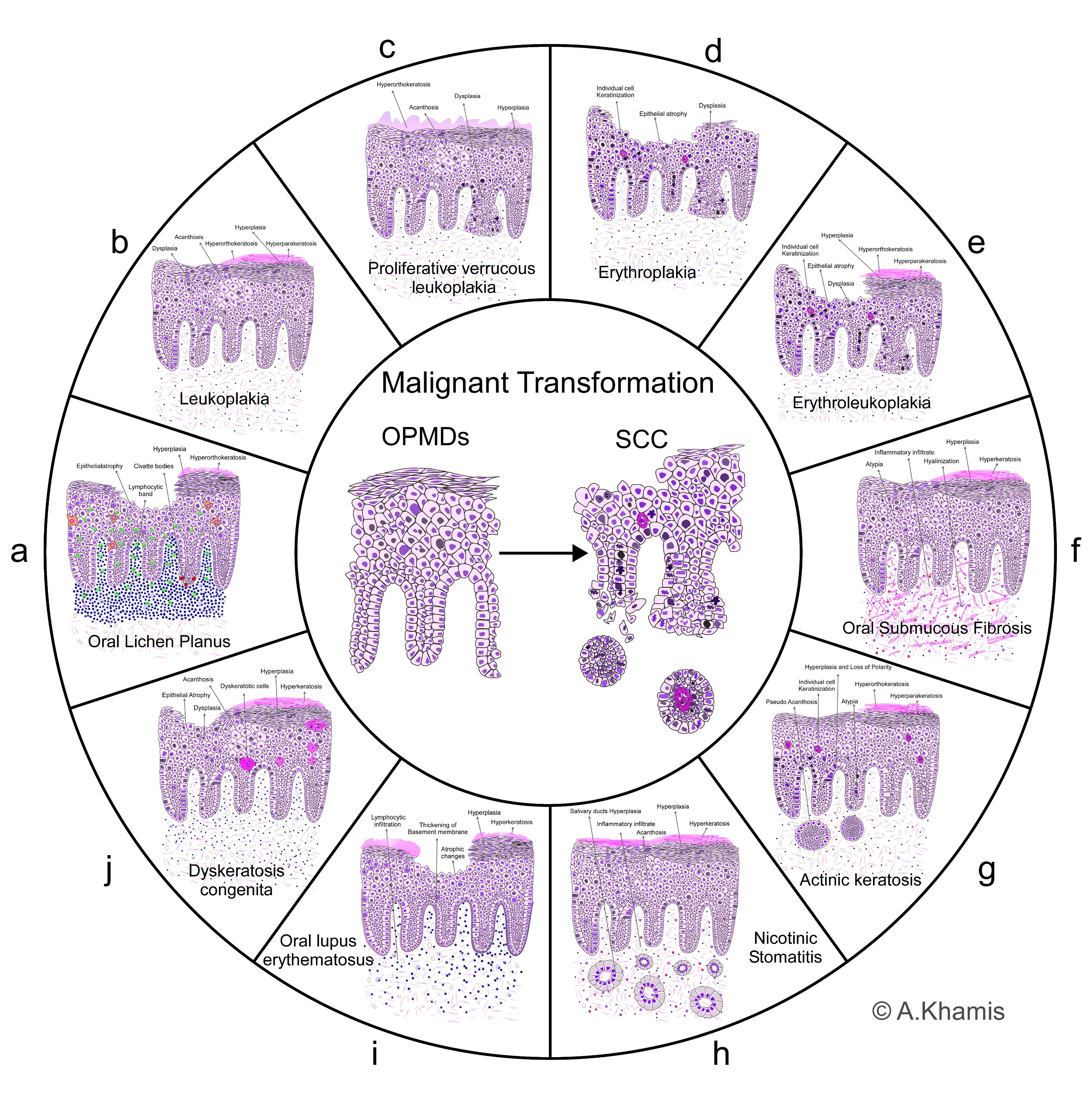This detailed medical diagram illustrates the biological processes involved in malignant transformation. Set against a white background, the circular chart is trimmed in black and divided into sections labeled from A through J. Each section displays an image of a cell, all colored in shades of light purple, representing various stages or types of cellular disorders. At the center of the circle, there are two organisms labeled "OPMDs" and "SCC," denoting the progression from oral potentially malignant disorders to squamous cell carcinoma, underlined by the phrase "Malignant Transformation" in black writing.

**Section Breakdown:**
- **A**: Oral Lichen Planus
- **B**: Leukoplakia
- **C**: Proliferative Verrucous Leukoplakia
- **D**: Erythroplakia
- **E**: Erythroleukoplakia
- **F**: Oral Submucous Fibrosis
- **G**: Actinic Keratosis
- **H**: Nicotinic Stomatitis
- **I**: Oral Lupus Erythematosus
- **J**: Dyskeratosis Congenita

This diagram appears to be used for educational or diagnostic purposes, potentially in the fields of oral pathology and oncology, highlighting different types of oral lesions and conditions that could lead to or indicate malignancy.